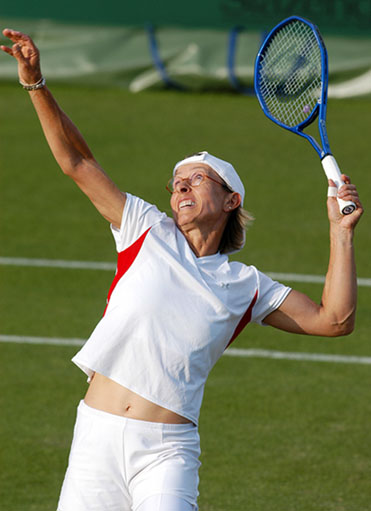In this image, we see a detailed depiction of an outdoor tennis court set under the bright midday sun. The surface is a flat, grassy field with various colored lines painted across, indicating it's a well-maintained sports arena. Towards the top of the image, a tarp is visible, adding context to the setting as perhaps a professional or semi-professional environment. Centrally framed is a female tennis player in action, captured mid-motion, suggesting she is about to hit a tennis ball. 

She is dressed in white shorts and a white short-sleeved, v-neck shirt with red side panels. She also sports a white baseball hat worn backward and red-framed eyeglasses. Her tennis racquet, featuring a white handle and blue frame, is gripped firmly in one of her raised hands. Her gaze is directed upward, focusing intently on something out of the frame, likely the ball. Behind her, slightly out of focus, are white lines marking the boundaries of the court and what appears to be a net, reinforcing the setting as a tennis court. The scene is vibrant with colors including green, white, red, blue, tan, dark green, and gray, all contributing to the lively atmosphere of this athletic moment. There is no text present in the image, allowing the detailed elements and the dynamic posture of the player to take center stage.